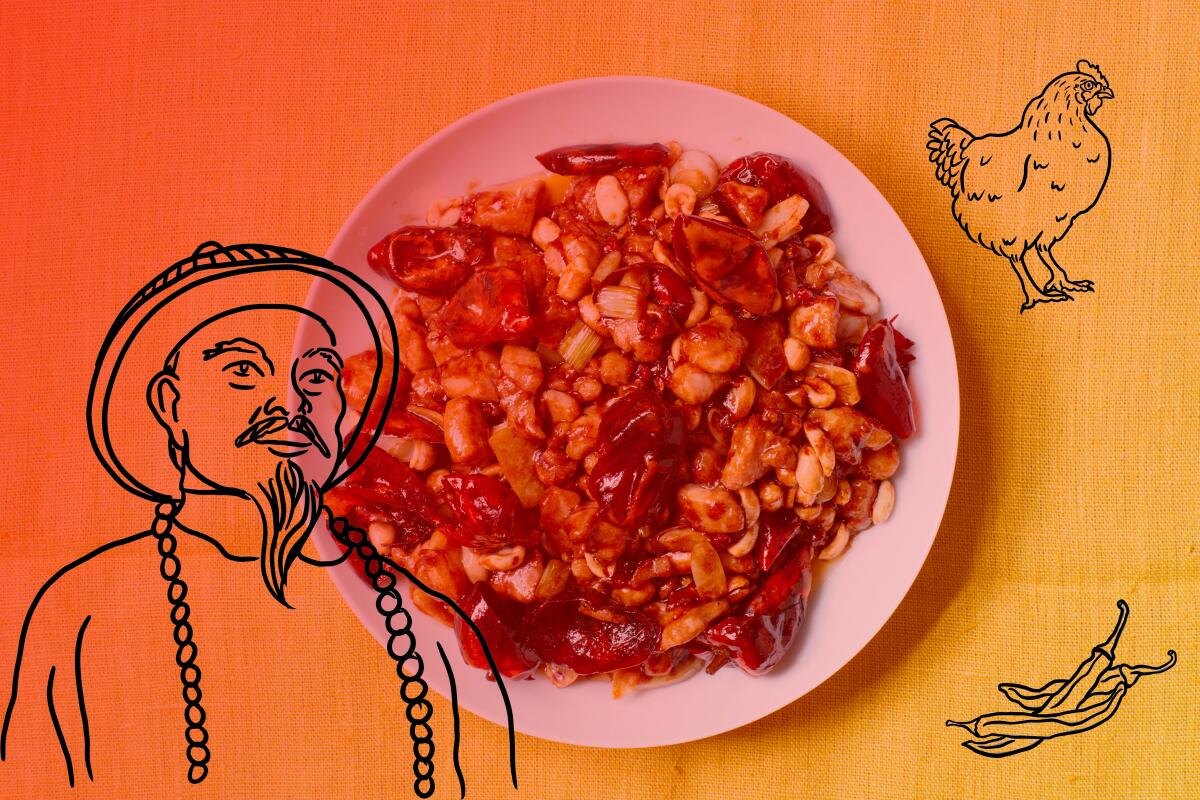This image showcases a vibrant culinary dish against an orange-yellow ombre background, presumably a tablecloth. The central white dish contains a hearty stew-like mixture, prominently featuring finely chopped chicken, red and yellow peppers, and possibly bits of celery or other vegetables, all bound together by a thick, savory sauce. The visual composition further includes overlaid cartoonish graphics: a silhouetted figure resembling a traditional Chinese man with a long beard and hat on the lower left, a chicken in the upper right corner, and peppers in the lower right corner. This meticulous presentation implies the dish is likely of Chinese origin, focusing on chicken and peppers, and could be intended for an advertisement or restaurant menu, even though there is no accompanying text.